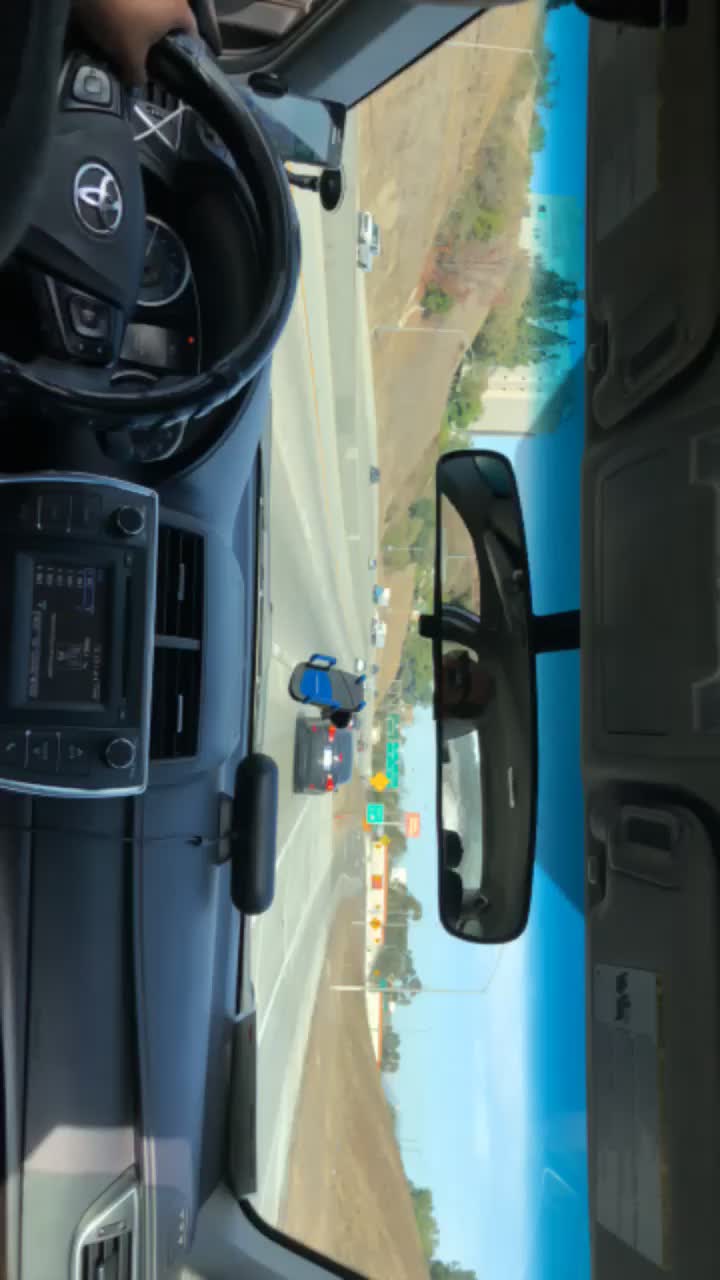A photograph taken from the interior of a car driving on a road, currently rotated 90 degrees to the right, reveals a detailed view of the dashboard and beyond. The scene, captured from the inside of a dark interior Toyota, shows the steering wheel with a prominently displayed Toyota logo positioned in the top left corner of the image due to rotation. A hand can be seen gripping the left side of the steering wheel. Behind the wheel, the speedometer is clearly visible, while the center console houses a media section with a radio adorned with a silver outline, flanked by two air conditioning vents above it.

Additional interior elements include a tablet-like device mounted in the center of the windshield, a fuzzbuster on the dashboard, and a suction cup cell phone holder on the window. The rectangular rear-view mirror, situated on the right side of the rotated image, reflects the driver wearing sunglasses and sporting short hair. The interior is primarily gray, with varying shades for different components, including light gray on the dash and darker gray around the AC vents.

Through the windshield, a clear view of the road shows a gray cement surface with a blue car in the right-hand lane bearing a white license plate. The road is flanked by dirt hills with sparse vegetation on both sides, and cars traveling in the opposite direction can be seen on the left side beyond a Jersey barrier. In the distance, a set of green highway signs and an orange diamond sign are visible, though the text is too distant to be legible. The road scene also includes an off-ramp leading to a white store with orange accents on the right side and a large white building beyond a steep hill on the left. The overall photo captures the essence of daytime driving on an American freeway, complete with the typical visual elements and a blue sky overhead.